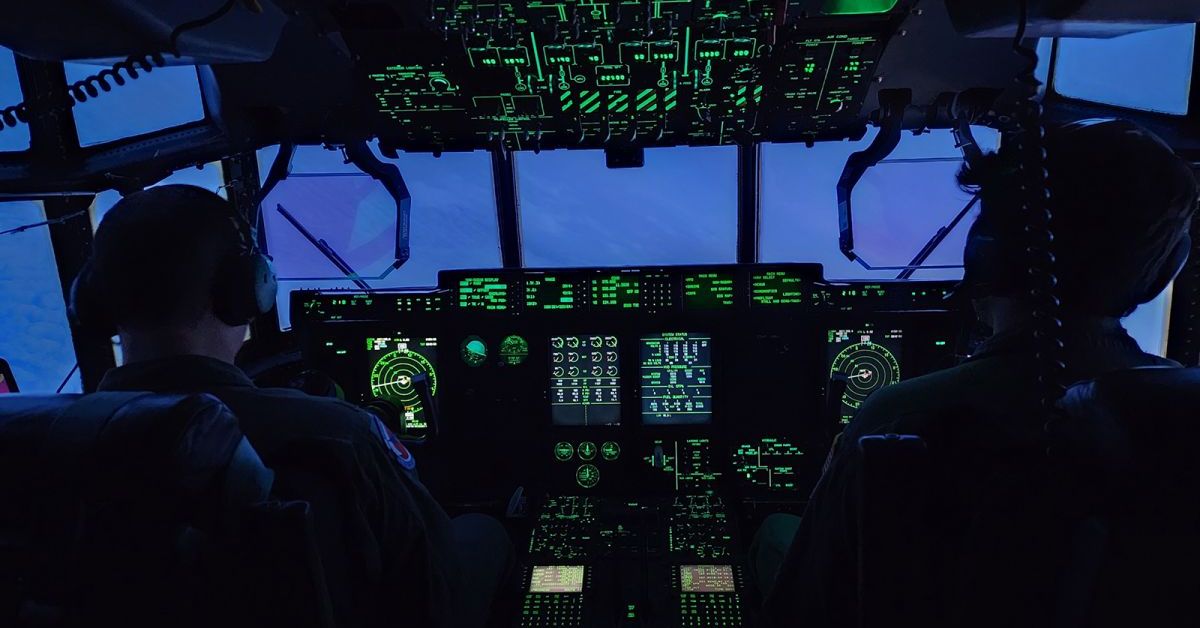The image depicts the interior of a jetliner's cockpit in flight, captured in a horizontal-rectangular shot. Framed from behind, the scene features the backs of two pilots' heads, distinctly positioned with the pilot on the left and the co-pilot on the right, both wearing communication headsets. The cockpit is awash with the glow of illuminated instruments, presenting a complex array of controls and displays. The primary instrument panel, as well as additional controls located above the windshield, are vividly lit, primarily with green reflective lights, contributing to the cockpit's intricate and high-tech ambiance. The scene outside the windshield is shrouded in the deepening hues of twilight or early night, casting a pretty purple color across the sky. The pilots' windows extend around to the sides, enhancing their visibility. Prominent features like a windshield wiper and various hanging instruments are also visible. The cockpit boasts a glass cockpit setup, featuring modern LCD or CRT displays that present crucial flight information, including engine conditions and speed, as well as radar data prominently displayed at the foremost point. The high level of detail in both the cockpit’s illuminated controls and the external twilight sky creates a captivating contrast.